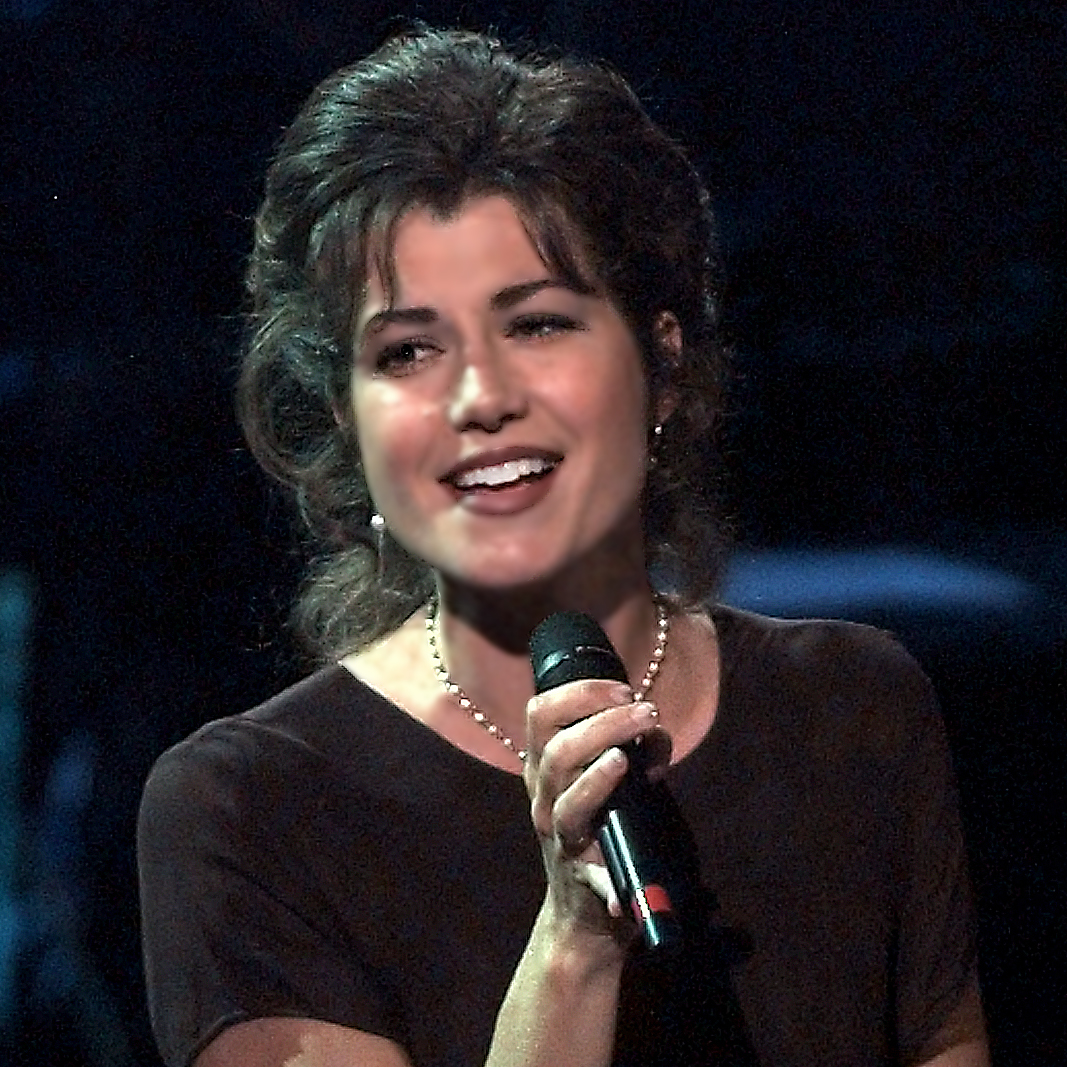The image portrays a woman with distinctive 90s-style voluminous hair, darker in color and quite shiny. She has well-done makeup with matte finishes and dark red lipstick. The woman is smiling while singing or speaking into a black microphone, and she is looking slightly off to the side. She is wearing a brown blouse or t-shirt and accessorizes with earrings and a necklace that appears to be made of diamonds or pearls. The backdrop is very dark, suggesting a stage-like setting, illuminated by subtle blue lighting near her shoulder. The shot focuses on her chest up to her head, with no visible text or words in the image. Prominent and shiny lighting emphasizes her hair, and the colors present in the photo include black, silver, light blue, red on the microphone, and the brown of her shirt. The setting is likely indoors.